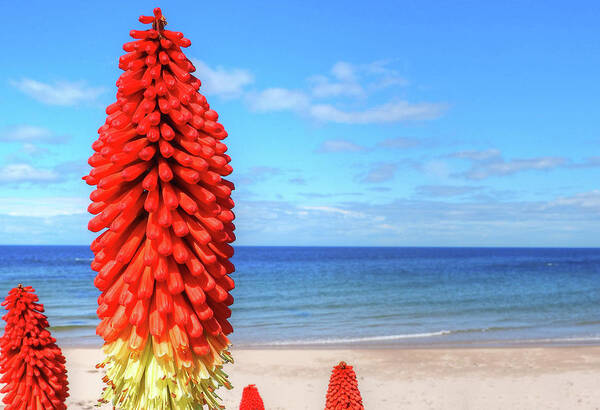This photograph captures a serene beachside scene under a partially cloudy, blue sky. The foreground features an impressive close-up of a large flowering tree. The tree displays stunning red rod-shaped seed pods, arranged in cone shapes, each cluster seemingly large and numerous. At the base of these clusters, the seed pods burst into yellow flowers, extending tendrils tipped with red nubs. The backdrop of the image reveals the soothing sand shoreline and clear, blue water of the ocean, creating a tranquil and picturesque setting.